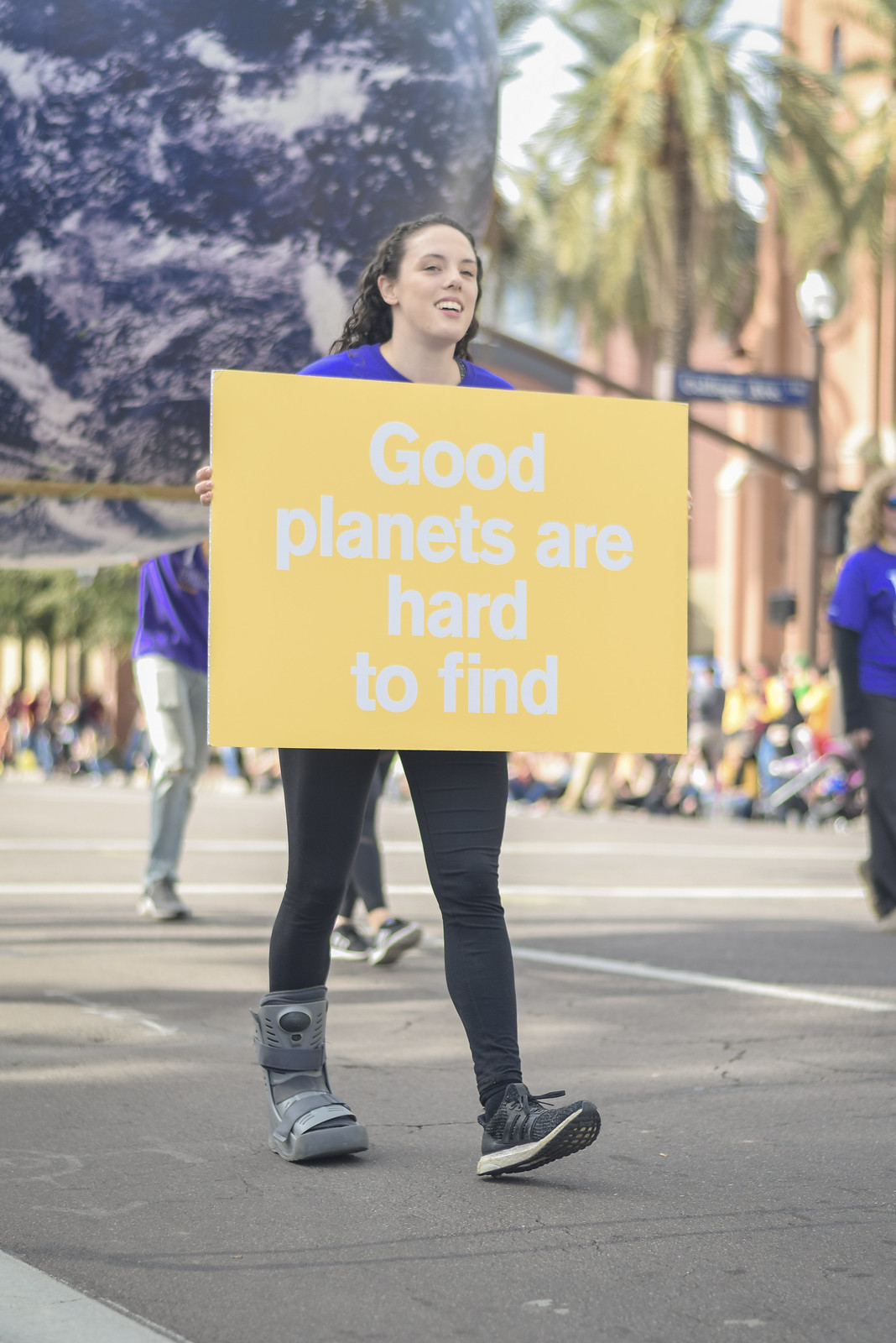This portrait view of a girl walking down a street captures the essence of a lively parade focused on environmental awareness. She holds a prominent yellow sign with white text reading "Good planets are hard to find," covering her torso from the chin to mid-thigh. Her attire includes a blue shirt, black leggings, a black sneaker on her right foot, and a gray walking boot on her left foot, suggesting dedication to the cause even while possibly nursing an injury. She has curly brown hair worn down.

The backdrop is vibrant with details indicating a warmer climate, likely California, as evidenced by palm trees and a blue street sign on a gray post. To her left, another woman dons a blue shirt and black pants, while a globed figure emerges in the upper left-hand corner, possibly carried by another participant. Blurry figures populate the background, some standing, some sitting, accentuating the parade atmosphere. The street is marked with white lines on the pavement, further cementing the scene as a bustling public event.